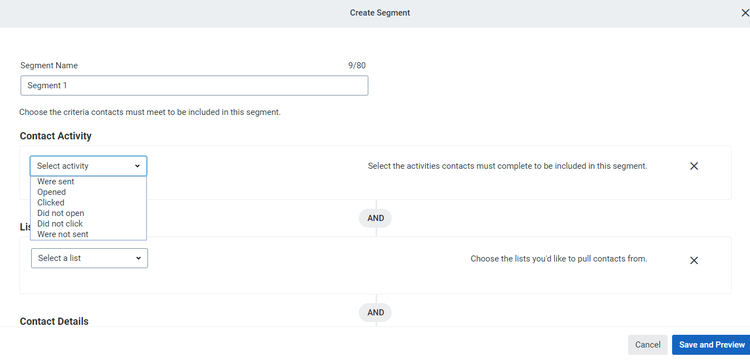The image features a user interface for segment creation, presumably within a digital marketing tool or CRM system. At the top of the interface, centered within a gray banner, is the title "Create Segment," accompanied by a small 'X' icon in the top right corner for closing the window. The main body of the interface is predominantly white.

On the left side, there's a section labeled "Segment Name" with an input field below it, allowing users to name the segment with up to 80 characters. Below this, instructions read, "Choose the criteria contacts must meet to be included in this segment."

A bold header titled "Contact Activity" allows users to select specific activities from a dropdown menu to filter contacts based on their actions. None of the activities are selected in the displayed image. This dropdown partially obscures another section that starts with an "L," likely referring to a "List" from which users can select entries.

Further down, a section labeled "Contact Details" is visible, but the image cuts off before revealing its contents. To the immediate right of the "Contact Activity" dropdown, there's an informational note clarifying that users should "select the activities contacts must complete to be included in this segment."

On the right-hand side, similar instructions are given for list selection: "Choose the list you'd like to pull contacts from," with an 'X' icon available for closing the list options.

The purpose of this user interface is not explicitly clear from the image, leaving it ambiguous whether it's part of a job-related tool, an app, or a website. The absence of an address bar and other identifying details suggests it could be a web application or a mobile app interface.